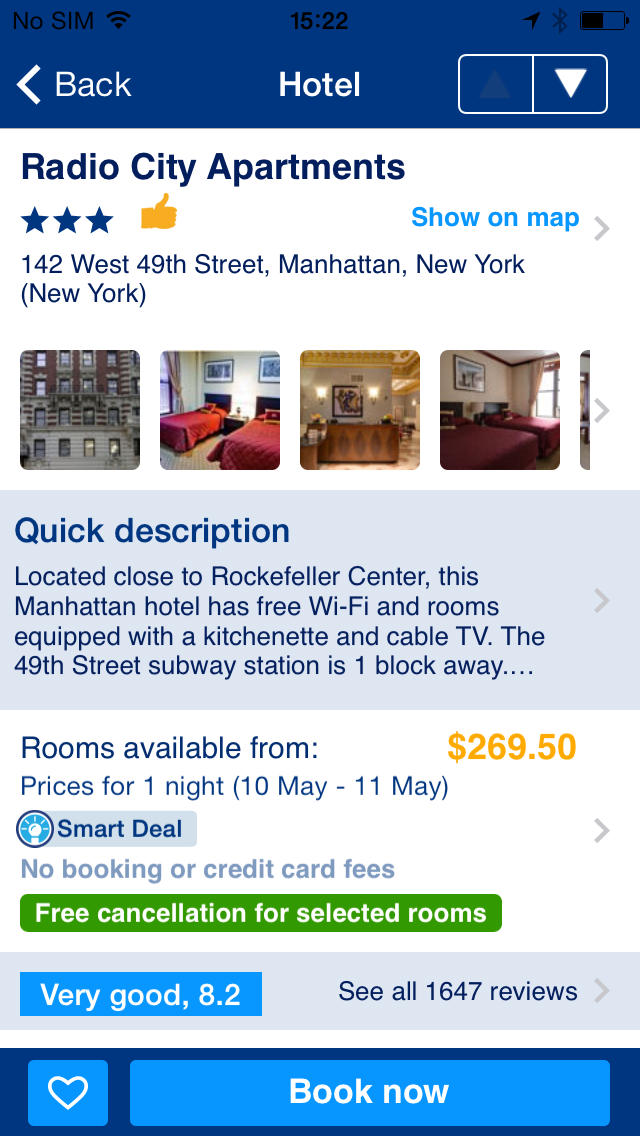Here is a cleaned-up and detailed caption for the image described:

---

This image is a screenshot from a cell phone. At the very top, a black status bar displays essential system information, including a "No SIM" message, Wi-Fi connectivity, the current time (15:22), active tracking, Bluetooth status, and a battery level just below half. Below this status bar is a blue navigation bar with white text reading "Back" on the left side.

In the center of the screen, the word "Hotel" is prominent, situated next to two icons on the right—one of which contains a triangle. Just beneath, we see a review for Radio City Apartments, accompanied by a three-star rating and a thumbs-up icon. To the right of the rating, a link saying "Show on Map" is available.

The address of Radio City Apartments is clearly listed: 142 West 49th Street, Manhattan, New York, New York. Below the address, thumbnail images of the apartment interiors provide a visual glimpse of the accommodations.

A boxed section beneath the thumbnails offers a quick description of the hotel: "Located close to Rockefeller Center, this Manhattan hotel has free Wi-Fi and rooms equipped with a kitchenette and cable TV. The 49th Street subway station is one block away." Following this, it mentions room availability and pricing: "Rooms available from $269.50 per night, for the dates 10th of May to 11th of May."

It highlights a "Smart Deal" with benefits such as "No booking or credit card fees" and "Free cancellation for selected rooms." Lastly, the review summary at the bottom displays a rating of "Very good, 8.2," based on "1,647 reviews."

A prominent, large blue button at the bottom of the screen urges users to "Book Now."

---

This detailed caption thoroughly describes the visual elements and text found in the screenshot, providing a comprehensive understanding of the image.